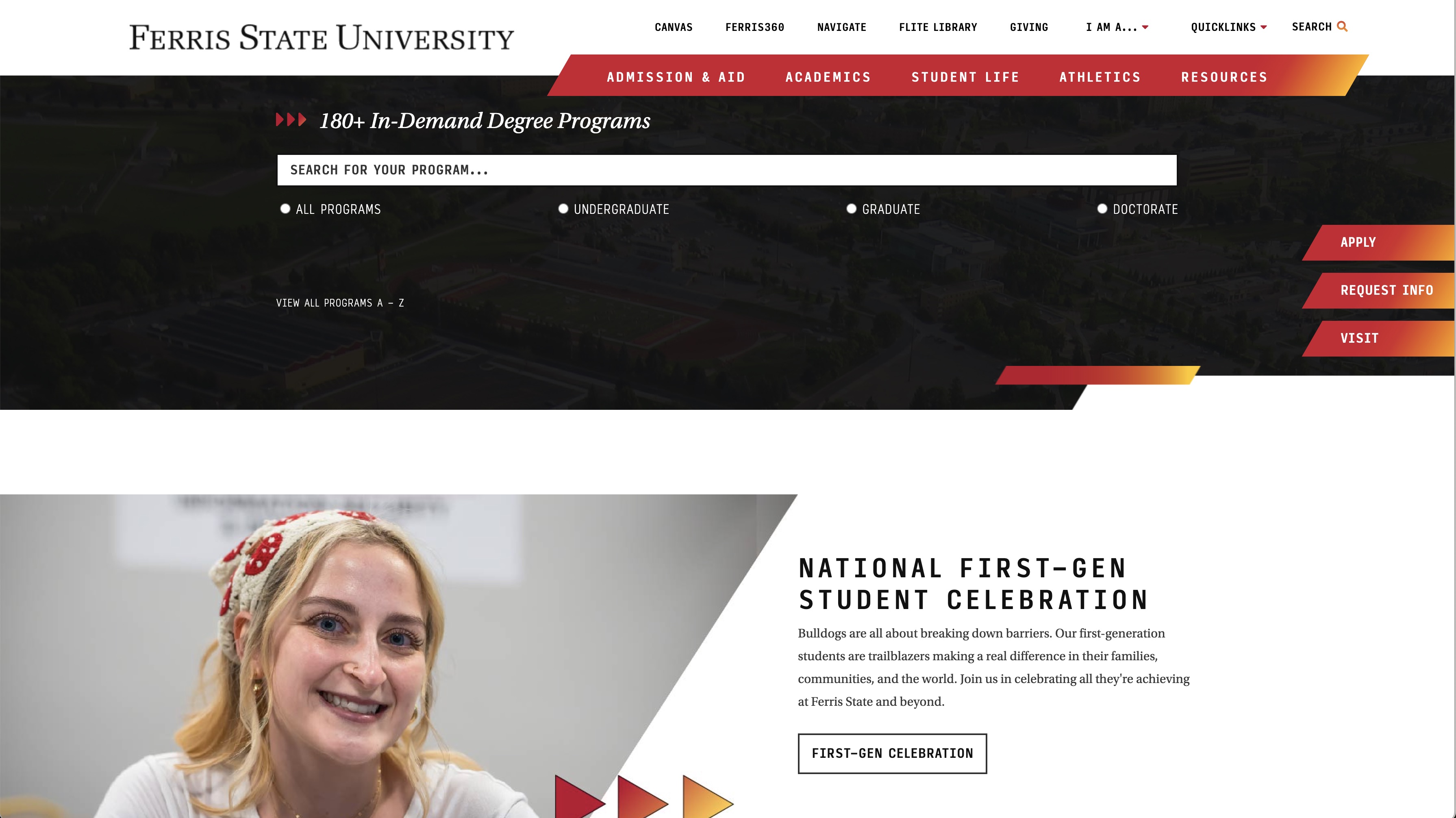This screenshot captures a section of the Beres State University website, prominently displaying various navigational elements and specific content. In the top left-hand corner, the title "Beres State University" is clearly visible, accompanied by a series of clickable options: "Careers," "Giving," "Navigate," and "Library." Directly below these options is a search bar, allowing users to look up specific programs.

On the right side of the page are additional links, including "Apply," "Request Info," and "Visit," facilitating easy access to important actions. Meanwhile, in the bottom left-hand corner, there is a visually engaging image featuring a smiling woman with light blue eyes, a fair complexion, and blonde hair, looking directly at the viewer.

Next to her image, there is a title reading "National First Gen Student Celebration" with a descriptive text below it. Additionally, there is a clickable button labeled "First Gen Celebration," directing users to more details about the event. Overall, this screenshot provides a detailed look at the homepage layout and resources available on the Beres State University website.